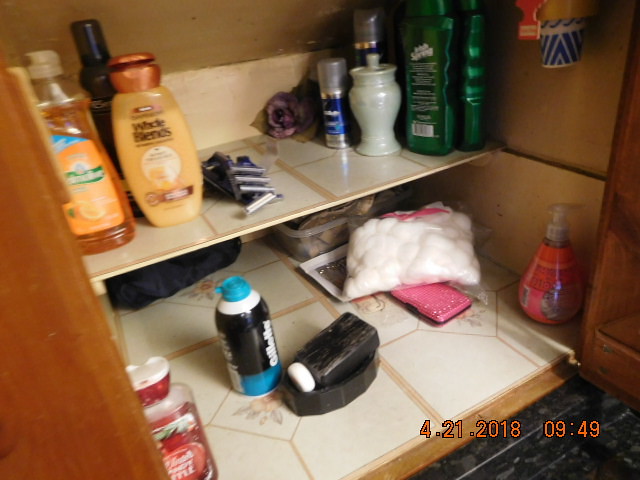A detailed photograph captures the interior of a bathroom storage cabinet, slightly tilted to the left, lending the shelves a diagonal orientation from the lower center to the upper right corner of the image. The cabinet's frame is composed of dark wood, creating a striking contrast with the white, tile-like shelves within. These shelves have a light-colored background, adding to the sense of depth and order.

On the bottom shelf, a collection of bathroom essentials are neatly arranged: several bottles of various cosmetics, including shaving cream, lotion, and hand soap with a pump dispenser. A shaving brush rests in a dish, accompanied by a bag of white cotton balls accented with pink labeling.

The shelf above houses an assortment of personal care items. To the left, an orange bottle of Palmolive dishwashing liquid stands out. Next to it, there is Whole Blends shampoo, a partially opened pack of razors, and in the back right corner of the shelf, a bottle of Iris Spring body wash. A deodorant and possibly a stack of Dixie cups are also visible in the upper right-hand corner of the cabinet.

At the bottom right of the image, against the dark wood floor of the cabinet, appears a time stamp: 4.21.2018, 09:49. This time stamp provides a temporal context for the meticulously organized, everyday items within the storage space.